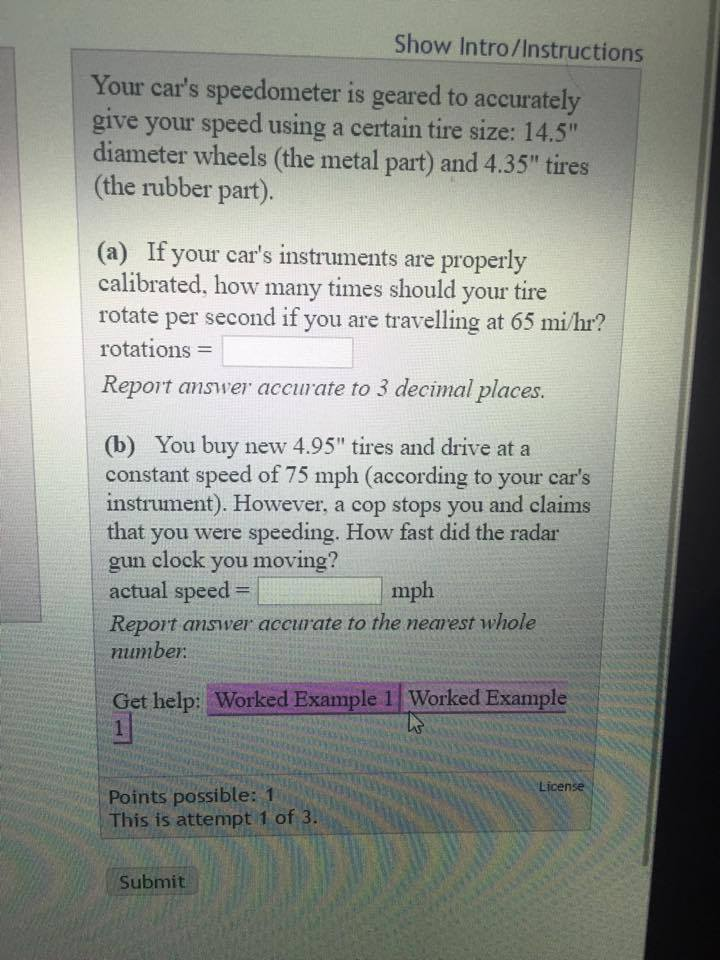In this image, we see a detailed display of a car's speedometer and odometer array on a screen. The speedometer is finely tuned to provide an accurate reading of the vehicle's speed, based on specific tire dimensions: 14.5-inch diameter wheels with 4.35-inch thick tires. For a vehicle correctly calibrated to these specifications, we can calculate that at a speed of 65 miles per hour, the tires should be rotating at a precise rate per second. The display poses an intriguing question: if a new tire is installed and the vehicle maintains a constant speed of 75 miles per hour, what speed is actually detected by a police radar gun? The image captures the technical details essential for determining the disparity between perceived and measured speed due to changes in tire size, illustrating the importance of proper calibration for accurate speed monitoring.